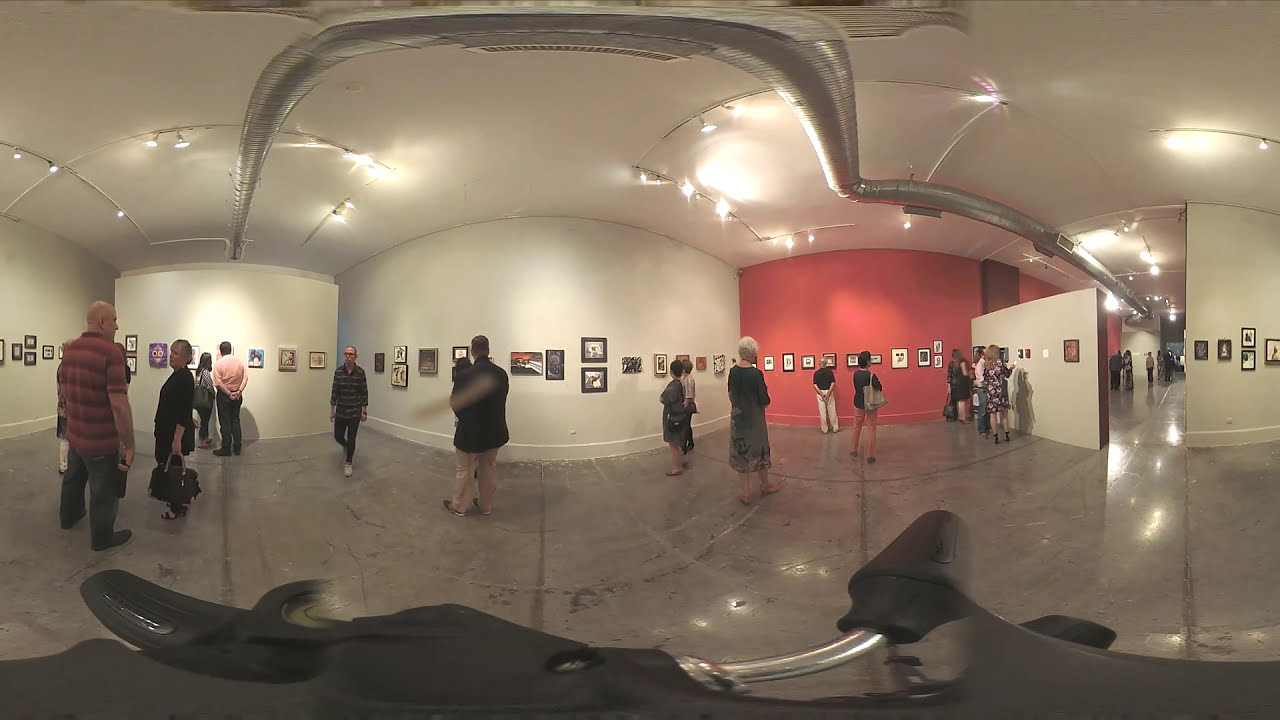The image captures a 360-degree view inside an art museum, showcasing a bustling gallery space. The walls of the display are staggered, predominantly white with sections of eggshell and a striking row of a light red or orange hue. The walls are adorned with numerous small, framed pictures, drawing the attention of many visitors scattered throughout the area. The floor beneath them is dark gray and reflective, adding to the modern ambiance of the space.

In the foreground, a rounded white wall features a multitude of small artworks, with clusters of people admiring them. To the right, a red-colored wall with a white partition leads to a hallway, where more people are seen immersed in the art. Farther back, additional groups continue to explore and appreciate the exhibits. On the left, another white wall partition in the middle of the room hosts more visitors who seem captivated by the displayed pieces.

The ceiling, peppered with lights and air ventilation piping, adds a functional yet industrial aesthetic to the gallery. The visitors, a mix of various ages, are thoroughly engaged with the art, with some intently staring at the paintings. Despite the distance, the artworks appear varied and small in size, contributing to the dynamic and vibrant atmosphere of the art museum.